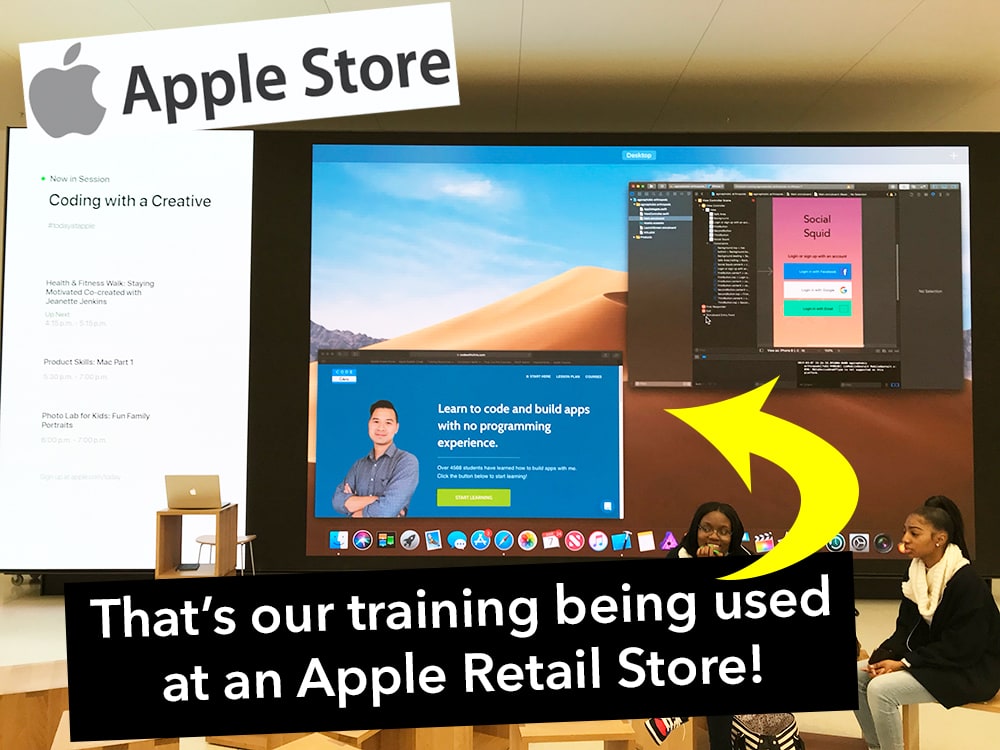In this screenshot, a large monitor dominates the scene, positioned in front of several seated individuals. To the right, two African-American women are visible; one is dressed in a black coat and leggings, while the other, partially obscured by a banner, wears a white scarf with her hair tied back. The banner, which predominantly covers the second woman, is black with white text stating that this is a training session being held at an Apple retail store.

Connected to the banner, an arrow points to a pop-up box on the upper middle left-hand side of the monitor. In this pop-up, a man, who appears to be either Hispanic or Caucasian, stands with his arms crossed against a blue background. The text beside him reads, "Learn to code and build apps with no programming experience," followed by additional smaller text and a green button, all written in white.

The background image on the monitor depicts a desert landscape with a hill of sand under a blue sky dotted with clouds. Another pop-up window is located on the upper right-hand side of the monitor, featuring the text "Social Squid" along with three buttons underneath. This section has a pinkish background, while the remainder of the pop-up is black with tiny text on the left side.

In the top left corner of the monitor, slightly tilted, a white banner displays "Apple Store" in black text alongside a gray Apple icon. Below this banner lies a white pop-up window resembling a coding interface, with some unrecognizable text and a creative label. Additionally, a plain brown wooden desk with a laptop sits to the right-hand side of this section.